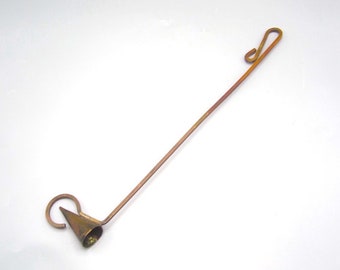This is a detailed photograph of a vintage candle snuffer, likely made from brass or copper, resting on a white surface that appears slightly shadowy around the edges. The snuffer features a long, slightly curved metal rod with a handle shaped like a paperclip at the end, designed for easy gripping. At the lower left-hand side, the rod extends to a metallic cone with an open base and pointed top, used to extinguish candle flames by depriving them of oxygen. The snuffer shows signs of age, with some patina and black stains, adding to its antique appearance. The simplicity of the white background, possibly for a product image, highlights the snuffer's rustic and vintage aesthetic.